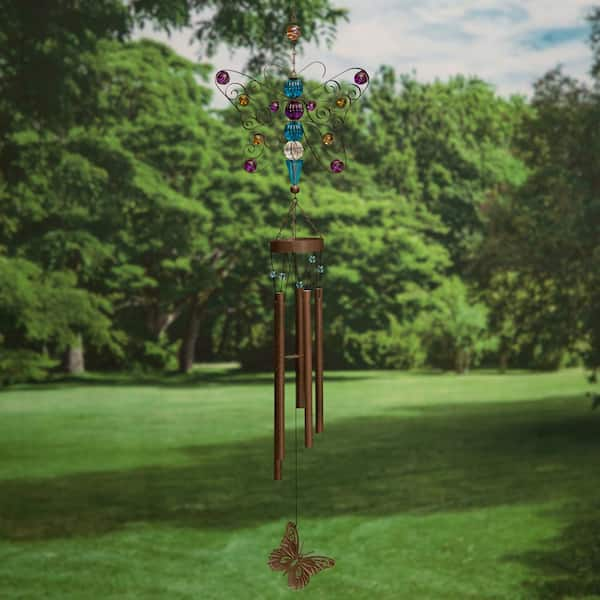The image features a copper-colored wind chime, prominently hanging from a tree in what appears to be a park or golf course with short, manicured green grass. The background showcases tall, vibrant trees with large green leaves. The wind chime itself is an intricate blend of copper elements and colorful beads. It consists of copper tubes attached to a top copper ring through blue beads. A copper washer or disc is seen in the center, preventing the pipes from rubbing against each other. Hanging from the bottom is a meticulously crafted copper butterfly. 

Further details include an upper butterfly figure made from a thin black wire frame adorned with blue, white, purple, and yellow beads. The butterfly features blue, purple, yellow, and pink stones, enhancing its wings. Two bent metal hoops form the antennae. A single chain, decorated with a gold bead, extends upwards from the butterfly, connecting the entire wind chime structure to the tree branch. Overhead, the sky is blue with scattered clouds, contributing to the serene backdrop.